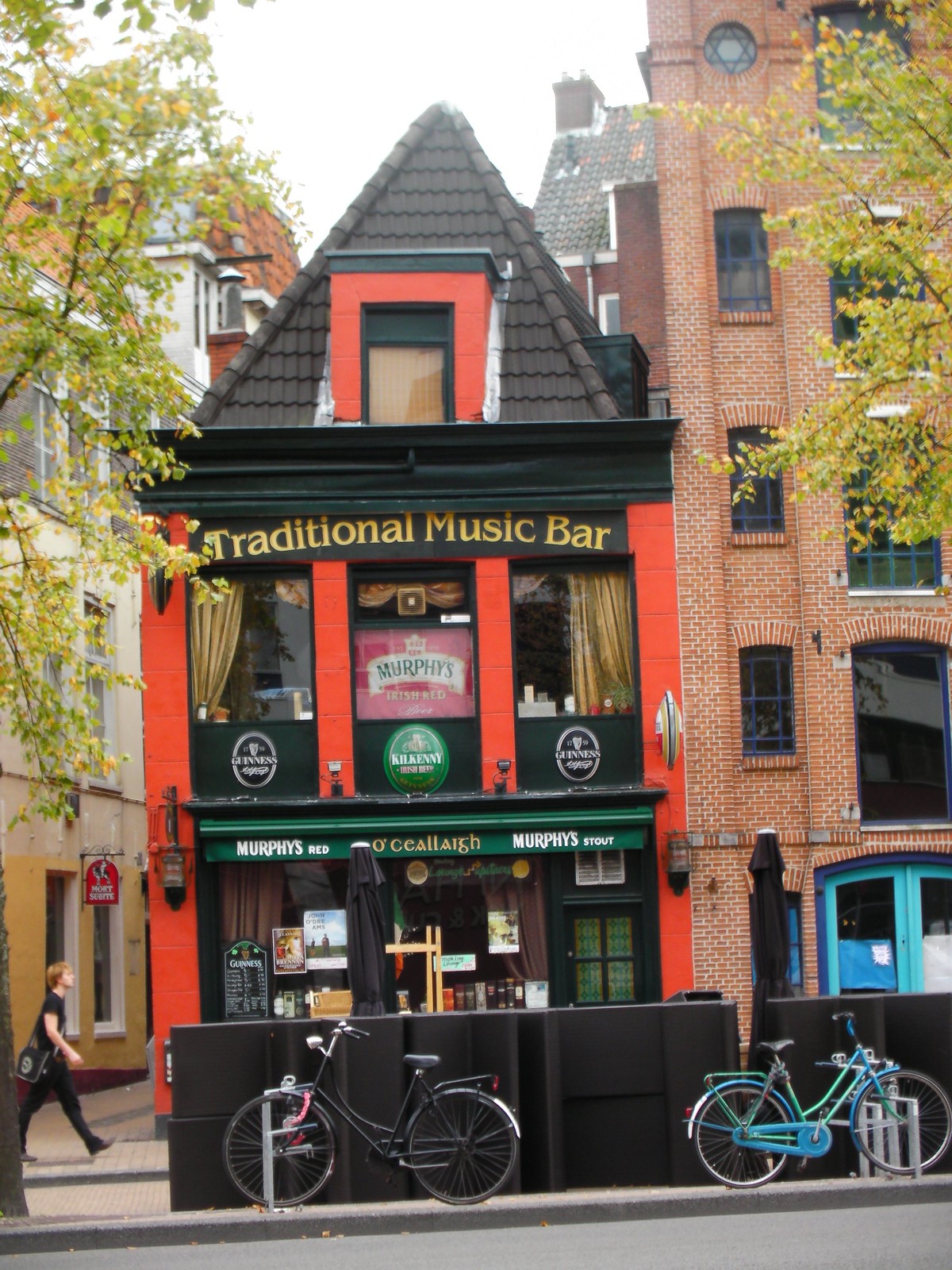The photograph captures a whimsical and uniquely styled pub named O'Callas, situated on a street flanked by larger, more nondescript buildings. Painted in striking hues of red, orange, green, and white, the pub stands out with its eye-catching design, including orange sashes and an attic window framed in orange, topped with a distinctive pyramid-shaped peak. Prominently displayed across the top of the facade is "Traditional Music Bar," indicative of its musical ambiance. Advertising for Murphy's Red and Murphy's Stout is visible both on the exterior and within the windows, which feature posters and a menu. Below, two bicycles—one black and one blue—are parked in front, while a person with red hair and dressed in black with a black shoulder bag is seen walking toward the entrance. The pub, adorned with lampposts and curtains, is nestled beside a brick building to the right and an office building to the left, creating a charming yet eclectic street view.